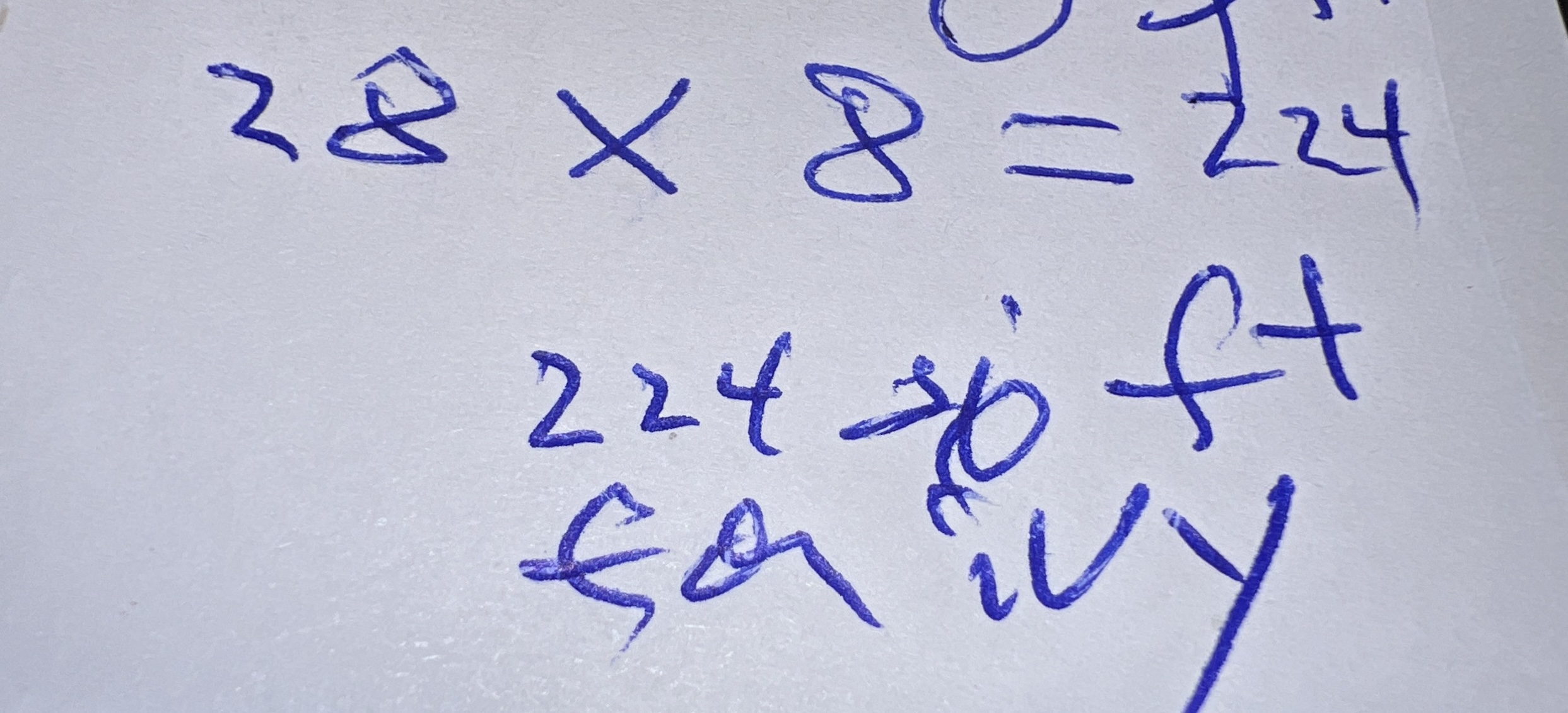This close-up image showcases blue text scrawled across a smooth white surface, capturing an intricate and somewhat smudged mathematical formula. The text appears relatively thick, though small areas of white show through, highlighting imperfections in the writing. The formula reads:

- "28 x 8 = 224" at the top, 
- Followed by "224 square feet."

Beneath this, there's a partially illegible word ending in "I-V-Y." The preceding letters are hard to decipher, with the first potentially resembling an "E" with a small tail, and the second resembling a circle with geometric appendages: a triangle pointing bottom-left and an upside-down L shape extending from the bottom-right.

Additionally, a small, cut-off portion of text is visible at the top right above the primary lines, appearing as part of a zero or O and a curved character nearby. The surface's ridges reflect faint highlights of light, particularly concentrated at the bottom center of the image, adding subtle depth and texture to the frame.